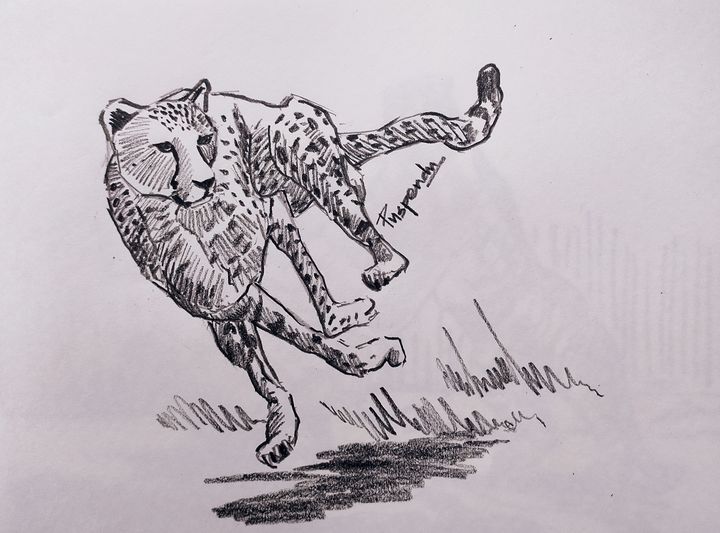This is a detailed pencil illustration in black, white, and gray, depicting a cheetah in mid-stride, running at full speed. The cheetah's body faces the viewer with its head slightly tilted to the right and downward, allowing visibility of both eyes and ears. All four of its legs are airborne, capturing a vivid sense of motion. The cheetah is covered in characteristic spots, with additional details such as visible whiskers and a black-tipped tail. Underneath the cheetah is a shadow, while in the background, squiggly lines suggest tufts of grass. The cheetah appears dynamic and lifelike, though the drawing has some imperfections. Between the cheetah's back leg and tail is a signature, difficult to decipher, possibly reading "P-U-S-P-E-N-D-N." The scene is set against a pale lavender background, emphasizing the depth and movement of the cheetah.